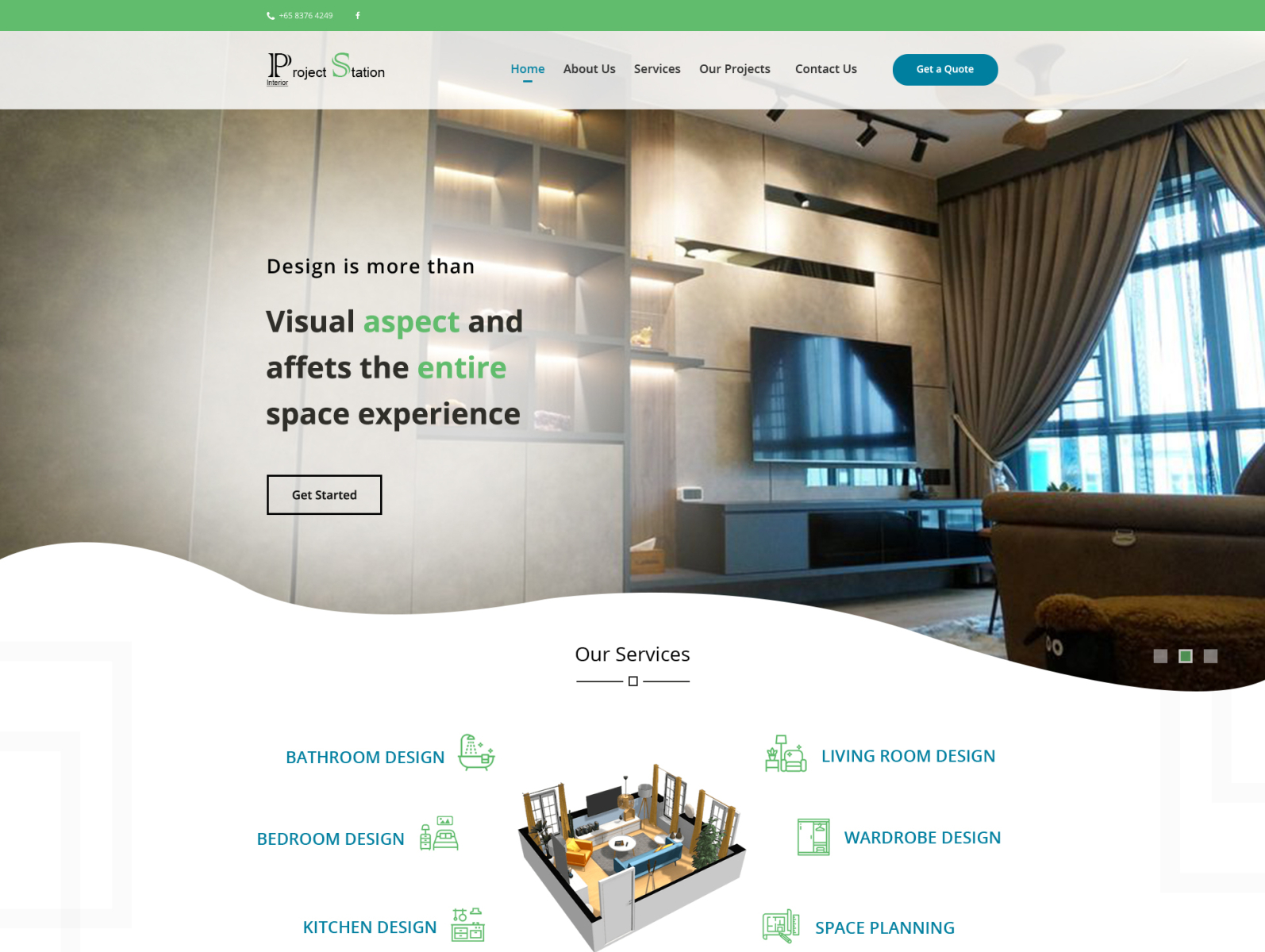Homepage Overview of Project Station Website

The homepage of the Project Station website features a top border in green, which includes a barely readable phone number next to a phone icon. The navigation tabs are: Home, About Us, Services, Our Projects, and Contact Us.

Beneath the top border, there's a prominent call-to-action bubble that reads "Get a Quote."

The central feature of the page is a stunning image of a living area showcasing an elegant entertainment center. The backdrop is a luxurious marble wall, complemented by a large window adorned with drapes and accentuated by track lighting. The living space also boasts a ceiling fan with an integrated light fixture, a stylish and comfortable chair, and what appear to be in-wall shelving units. These shelving units are configured as follows: a top space divided into two side-by-side compartments, followed by another open area with two sections below it.

Overlaying this image is the text: "Design is more than a visual aspect; it affects the entire space experience." Below this text is a prominent "Get Started" button.

Further down the page is a section titled "Our Services," which is divided into two parts:

- On the left: Bathroom Design, Bedroom Design, and Kitchen Design.
- In the center: An image of another beautifully designed living area.
- On the right: Living Room Design, Wardrobe Design, and Space Planning.